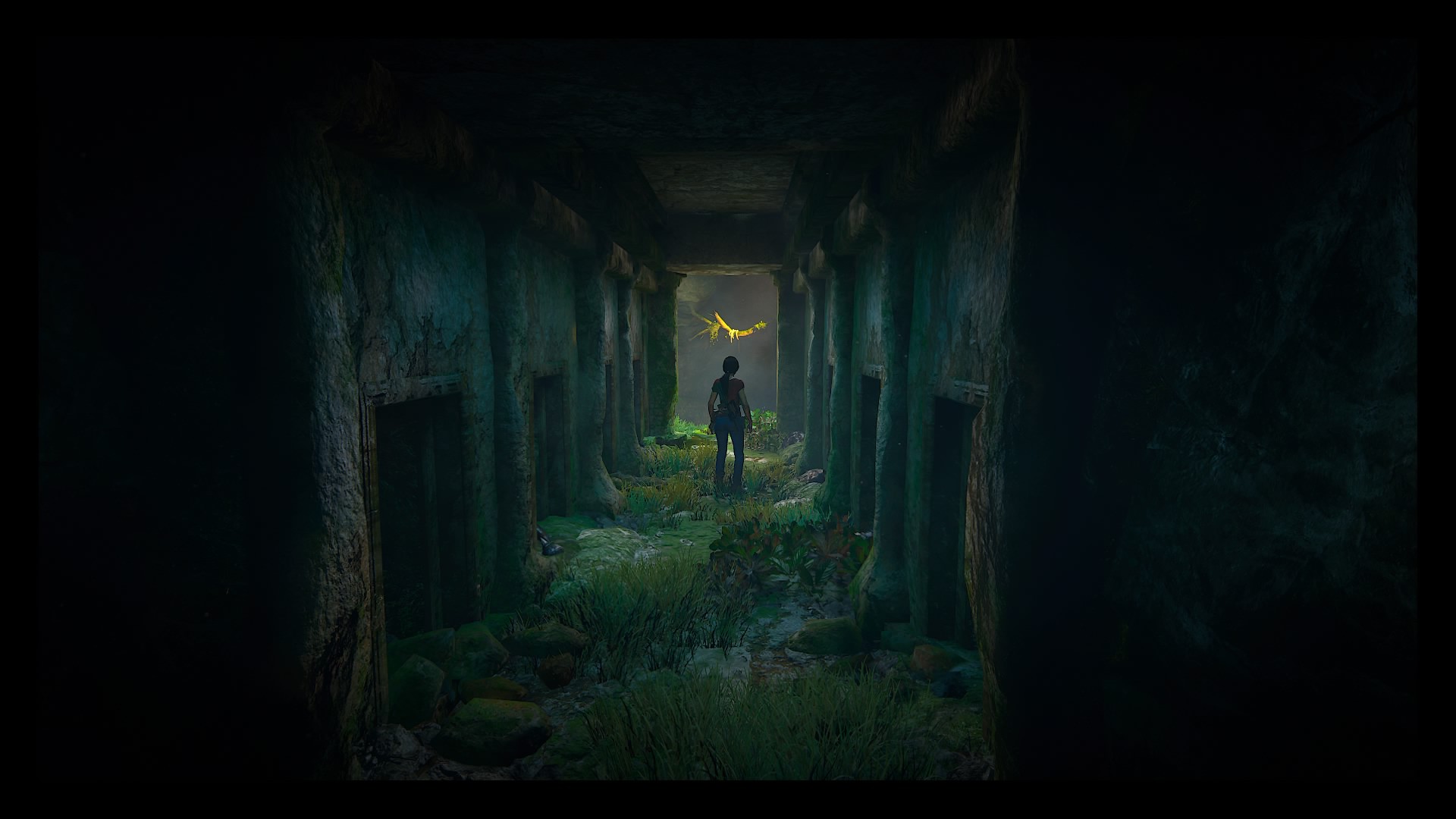In this image, presumably from a video game, a dark, narrow hallway stretches into the distance. The hallway features rugged stone walls on either side, adorned with patches of green grass and rocky surfaces covered in vibrant moss. The stonework displays a mix of white and brown hues, and some sections show small recesses where the stones have eroded. In the distant part of the corridor, a bright yellow branch or object stands out against the darker background. 

In the foreground, a character with blue jeans and a reddish shirt, their hair tied back in a ponytail, stands poised. The scene strongly suggests it could be from a modern Tomb Raider game or perhaps the Uncharted series, specifically the DLC featuring a female protagonist.